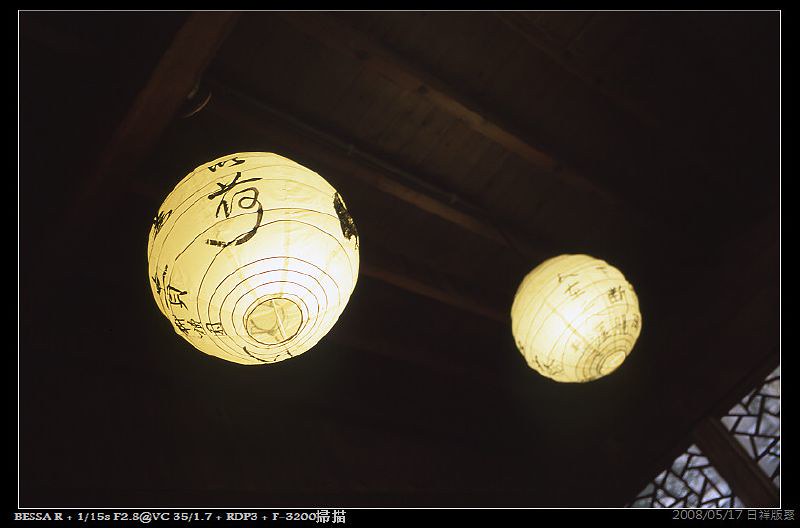This image captures a dimly lit room, likely within an Asian restaurant, featuring a rich brown wooden ceiling with beams, giving the space a warm, authentic ambiance. Dominating the scene are two glowing, yellowish-cream colored round paper lanterns adorned with black Japanese or Asian characters, serving as the focal point. The lanterns' glow reveals their internal spiral metal structures, adding to their intricate beauty. A stained glass window is visible in the lower right corner, contributing to the ornate details of the room. At the bottom of the image, a series of numerical and alphabetical figures including "BESA R.1", "3200", and other Japanese or Asian writings are visible, potentially indicating a catalog or professional photography information. The entire image is framed by a thin white line, providing a distinct contrast against the black background.